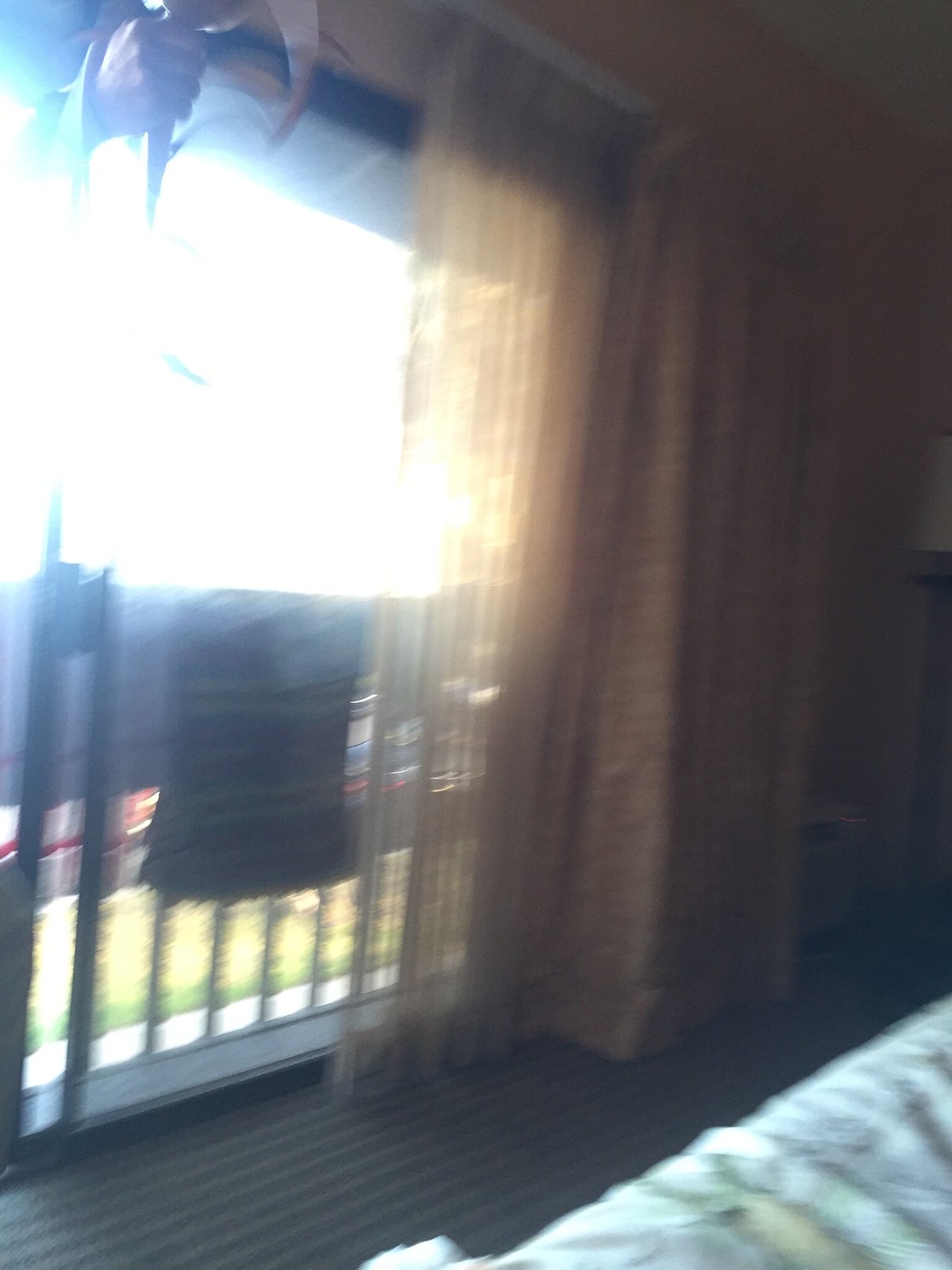The photograph depicts a blurry and possibly accidental shot taken from within what appears to be a bedroom or hotel room, looking out through a sliding glass door. The room itself features a tan to nearly orange curtain that is lighter and more translucent where sunlight filters through, casting a brighter light on parts of the scene while obscuring some details. Adjacent to the sliding glass door is a railing with clothes or towels hanging over it, drying in the daylight. Below, you see a brown floor and in the lower right-hand corner, there is a white blanket adorned with green and yellow patterns. A person's hand is visible in the upper left-hand portion of the image, though what they are holding remains unseen. Outside the glass door, there are hints of green, possibly grass or hedges, partially obscured by the bright sunlight. The image includes an orange-colored wall in the background, adding to the warm tones of the interior.